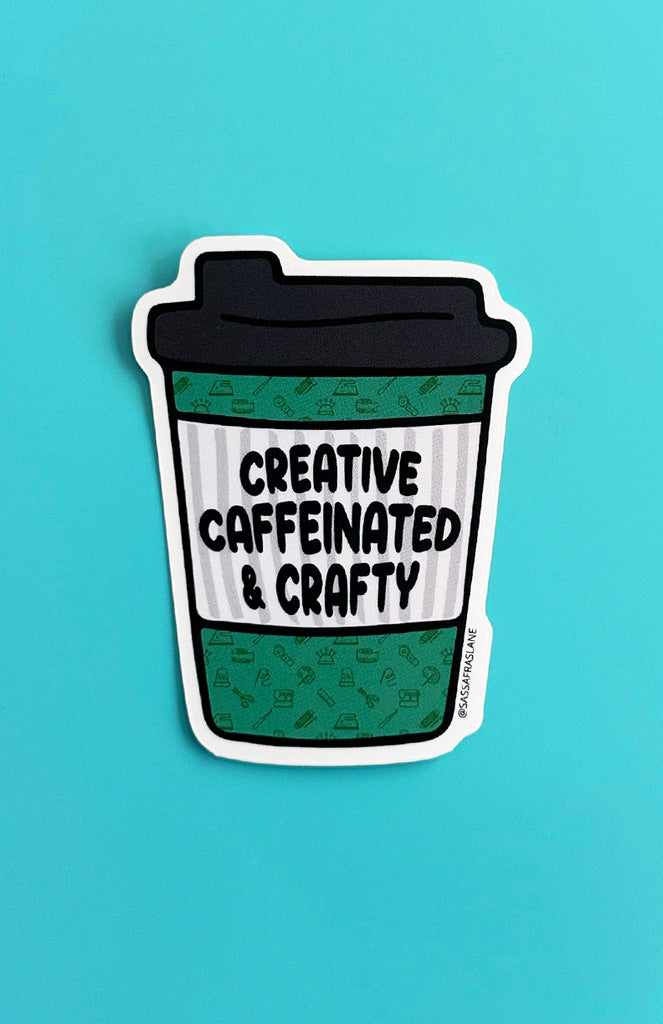This photograph captures a sticker sitting on a light blue surface. The sticker depicts a green paper coffee cup adorned with a black lid. The lid features a small spout at the top, characteristic of a typical coffee cup lid. The main body of the cup is green with black patterns and has a prominent white label. The label bears the words "CREATIVE, CAFFEINATED, and CRAFTY" written in bold black letters. The edges of the sticker have a white border, making it stand out against the solid baby blue background. The sticker appears to be designed for easy application, possibly on the side of a mug or another surface.